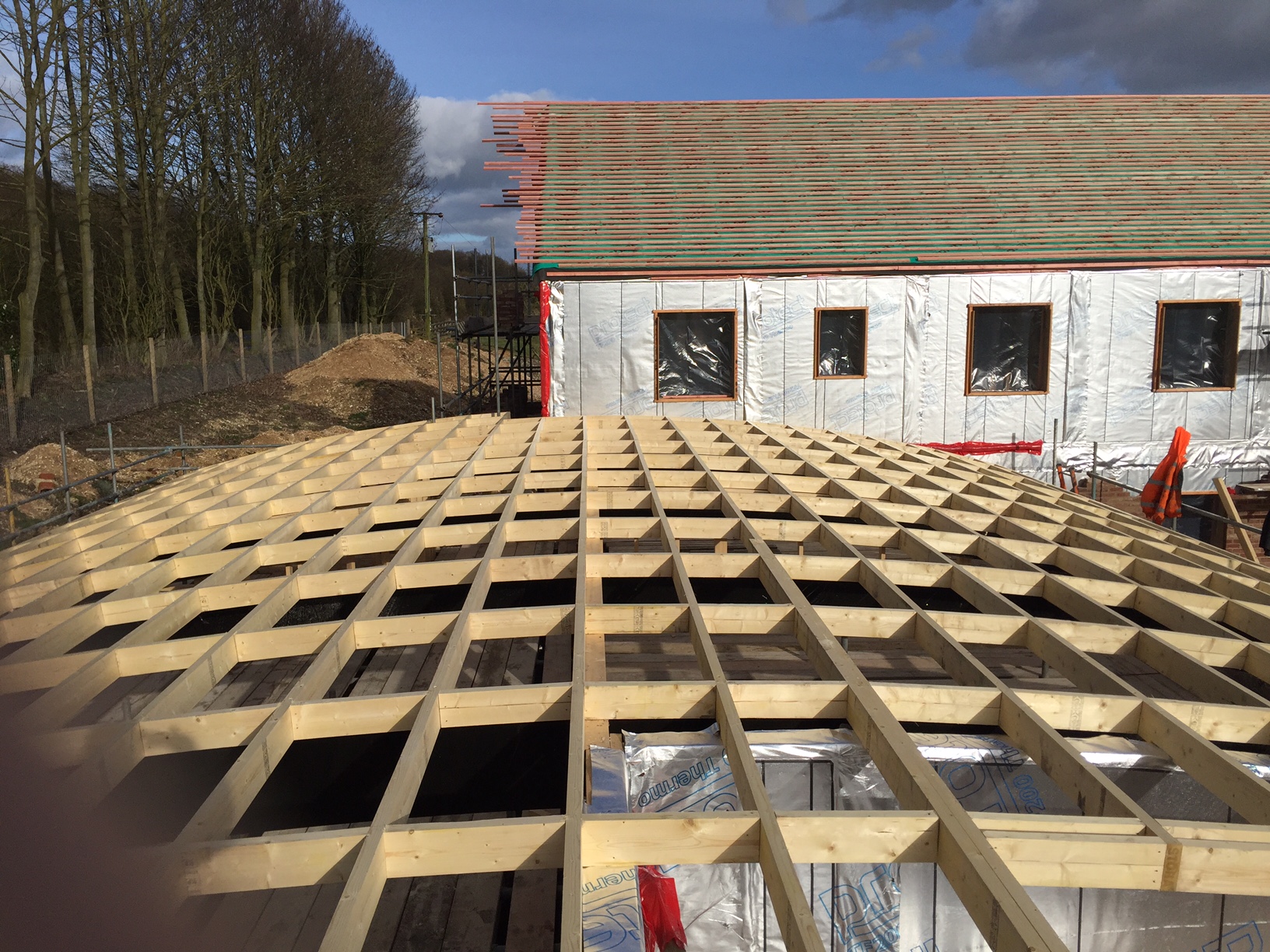The image captures an active construction site featuring multiple buildings at various stages of development. Dominating the foreground is an unfinished wooden roof structure with a slightly curved design, made of two-by-fours and two-by-sixes positioned at regular intervals. The photo appears to be taken from atop this roof, emphasizing its skeletal frame devoid of any finishing materials.

To the right, another building stands partly wrapped in silver insulation with pre-cut window spaces covered by plastic sheeting. This building, at least two stories high, features an incomplete roof and an external structure, possibly a fire escape or balcony, on the second level.

The left side of the image reveals a construction fence and a straight line of mature trees, separating the site from piles of excavated dirt that slope gently downhill. The entire scene is bathed in the angled light of early morning or late evening, adding depth and contrast to the image.